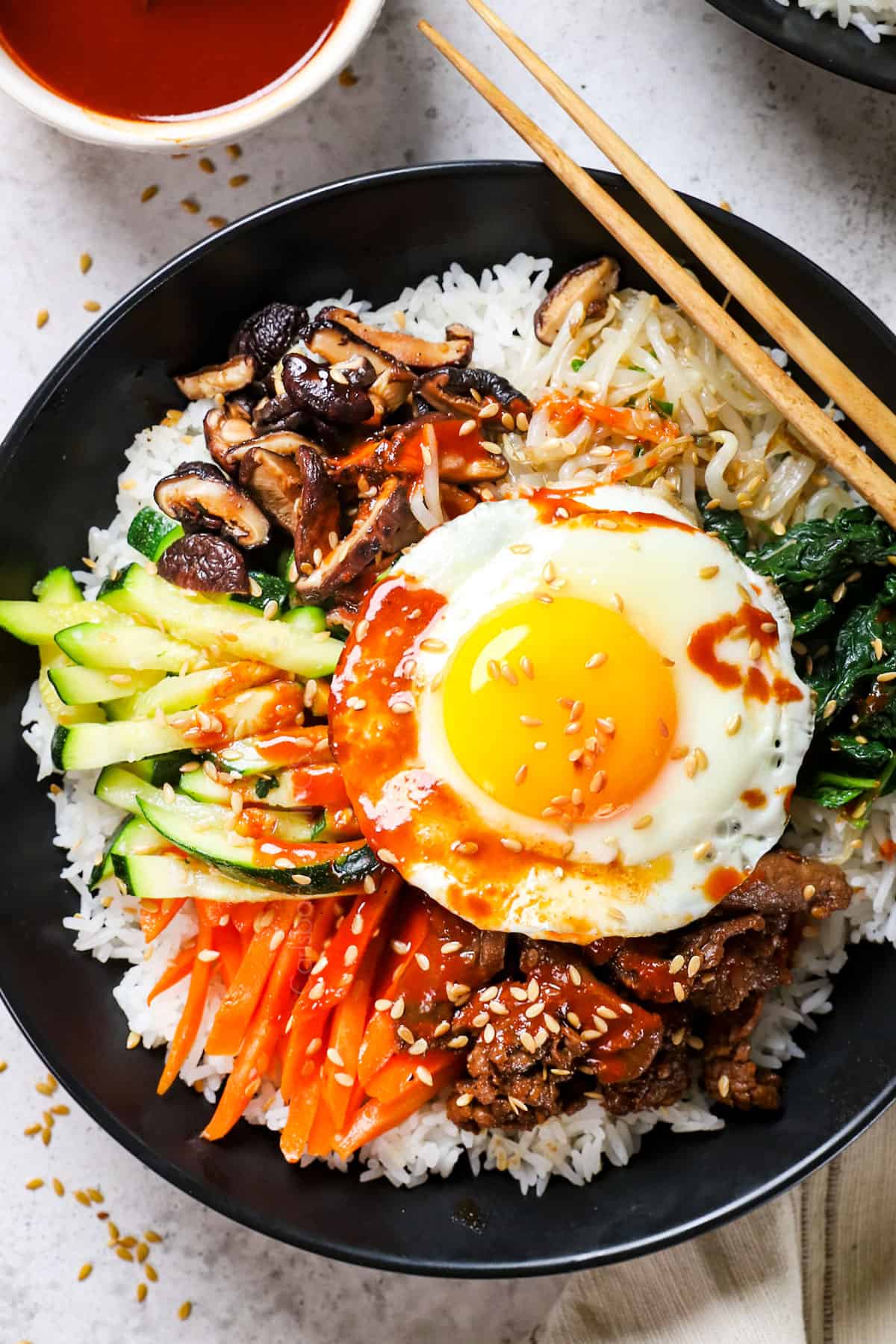The image depicts a beautifully arranged dish on a black, round plate, which rests on a marble countertop, likely an indoor setting reminiscent of a food blog or advertisement. The plate is centered in the frame, with the backdrop hinting at a marble backsplash. The culinary creation on the plate features a base of rice, adorned with an array of vegetables including carrots and cucumbers, along with greens that might be spinach. Mushrooms and a few noodles are also visible, lending texture and variety to the dish. Positioned prominently in the center is a sunny-side-up fried egg, its yolk vibrant and enticing. Surrounding the egg is a serving of beef, glistening with a soft sauce. The entire dish is drizzled with a red sauce that also appears in a bowl situated at the top left of the image. Completing the setup, two chopsticks are seen on the right-hand side of the plate, ready for use, emphasizing the dish's inviting presentation.